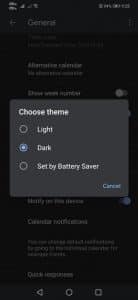This is a detailed screenshot of a mobile phone's settings section, specifically under the "General" settings. The background of the image is black, and although the background is quite blurry, the text remains clear and is displayed in white. The settings page features various sections, some of which include toggle options.

Overlaying the settings page is a gray pop-up box. The header of this box, also in white text, reads "Choose Theme." Below this header, there are three options aligned in a column with corresponding radio buttons. The first option is "Light," the second is "Dark," and the third is "Set by Battery Saver." The "Dark" option is currently selected, as indicated by the filled radio button.

At the bottom-right corner of the pop-up box, there is a "Cancel" button marked in blue. Additionally, the standard navigation bar at the bottom of the screen includes a backward triangle (back button), a circle (home button), and a square (recent apps button) arranged in a row.